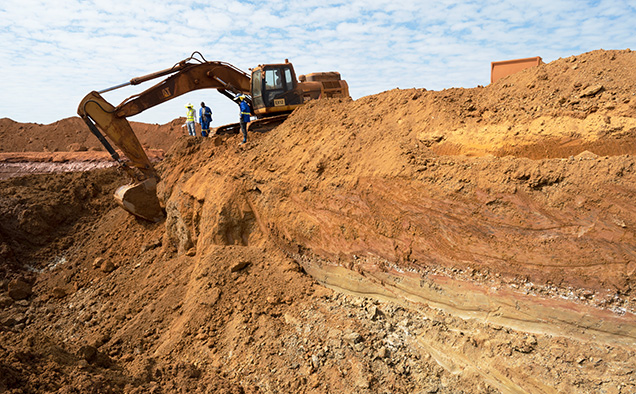In this photograph, a large yellow CAT-brand excavator is in the midst of a heavy excavation operation on a sunny day, indicated by the clear blue sky and puffy white clouds. The excavator is prominently positioned in the upper left corner, extending its bucket on a swing arm deep into a chasm of varying shades of tan and light red dirt, which appears to be primarily composed of red clay. The operator is visible through the machine's windows, actively manipulating the controls to dig and lift dirt and rocks, forming mounds of excavated material both in the background and foreground. To the right of the machine, three workers stand at the edge of the excavated area, observing the ongoing work. One worker is dressed in a yellow sombrero, yellow safety vest, and worn pants, while the second worker wears a blue vest and pants with a white undershirt. The third worker, positioned to the right of the excavator, wears a blue cap, blue vest with yellow safety stripes, gray or black pants, and sun protectors on his neck. The image captures the dynamic interplay of human and machinery involved in the earth-moving process.